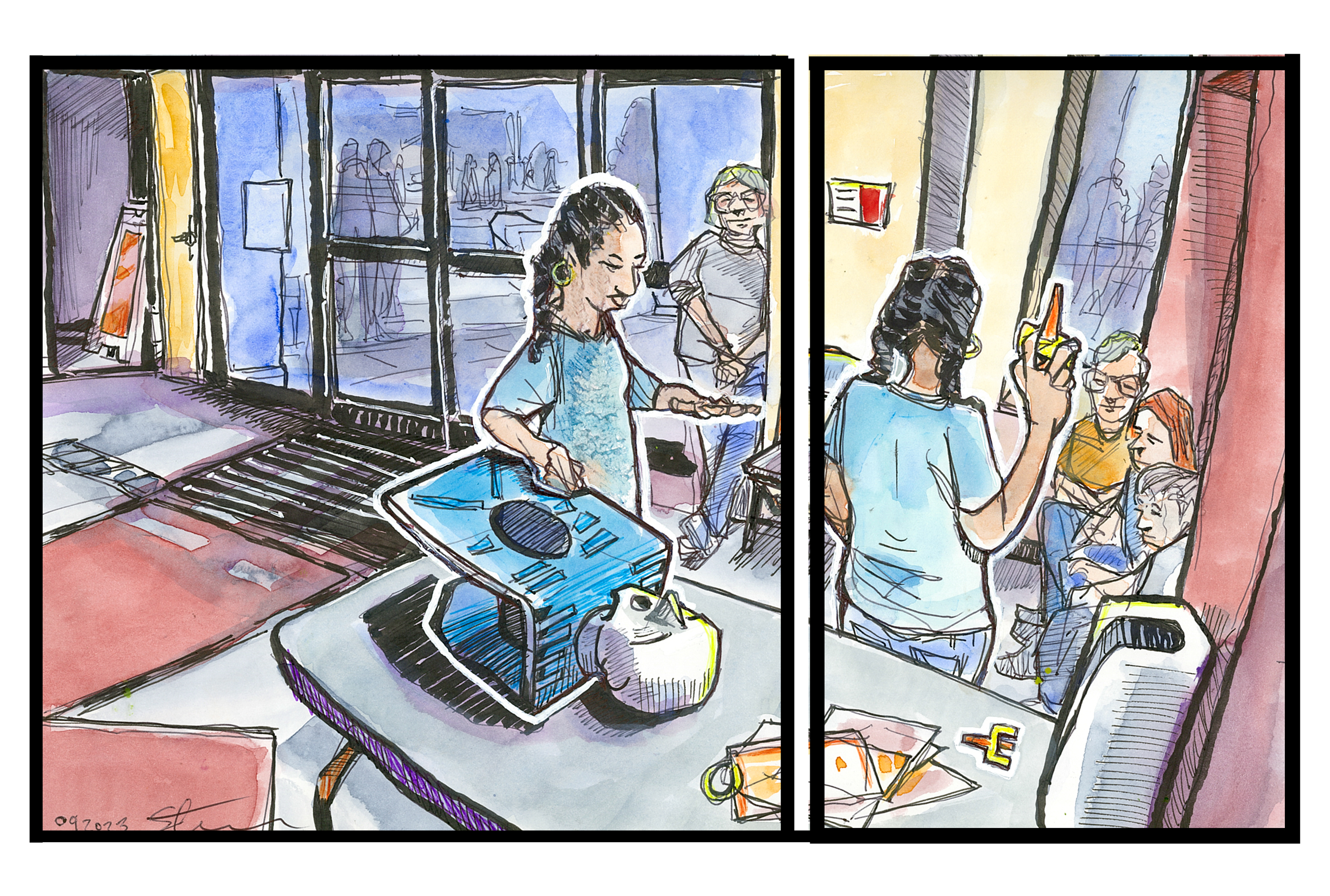In the vibrant, colorful comic-style drawing, we see a young Black individual with cornrows and a loop earring in their right ear, wearing a T-shirt. They are depicted in two panels, creating a split narrative. In the first panel, the individual rests their right hand on a blue rectangular device, standing near dual glass doors with a small caution sign. An older woman leans against the wall, observing, possibly her mother. In the second panel, the same individual, now seen from the back, faces three seated people, holding what appears to be a plunger-like object. The scene suggests a setting where the young adult might be operating a store or a service area, with colorful, expensive markers used in the artwork to enhance the lively and detailed environment. Various characters, including an older man in boxes, contribute to the dynamic scene.